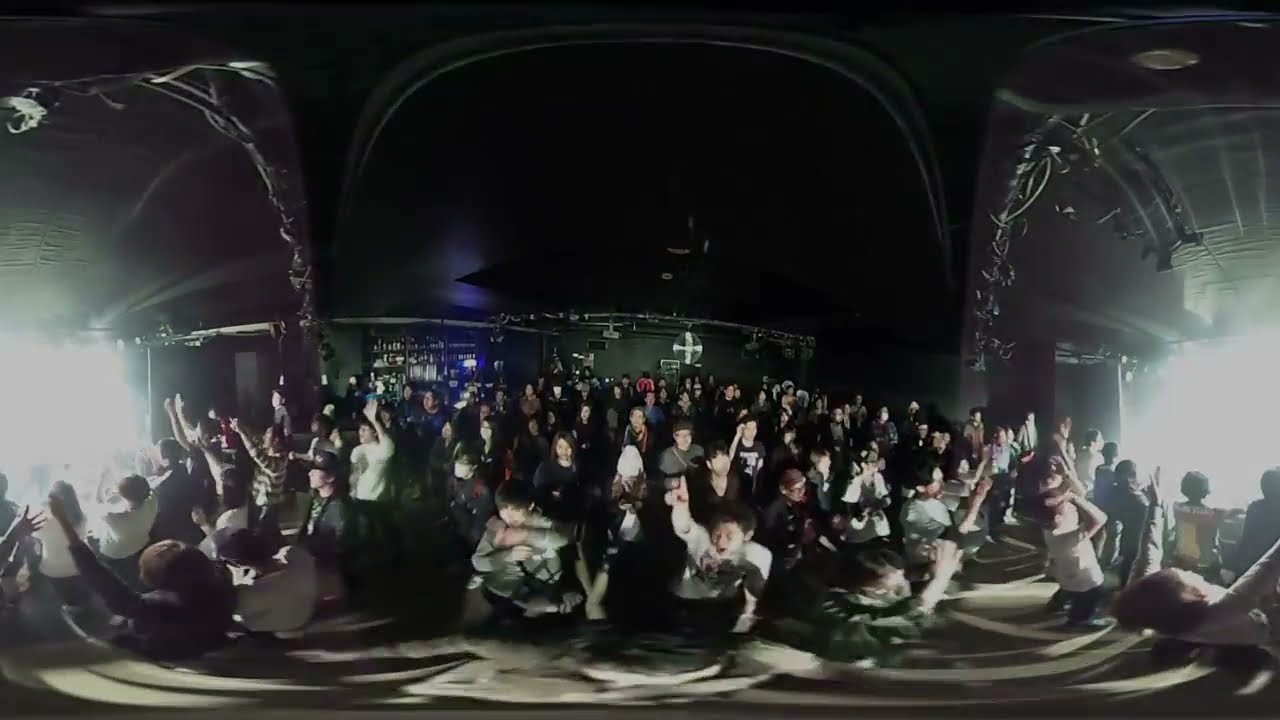The image depicts an indoor concert venue filled with a large, energetic crowd, their arms raised in excitement, some with pointer fingers up, reflecting the lively atmosphere. The picture is notably warped, possibly taken with a 360-degree camera, creating a curved and distorted view where the left and right sides mirror each other, capturing the concert action from both perspectives. In the far back, a wall with a greenish tint and a prominent white cross symbol stands out amidst the otherwise dark venue, with dim lighting accentuating the black, white, gray, silver, blue, and red hues throughout the scene. A bright, glowing light from the stage casts upon the audience, obscuring the musicians but highlighting the fervor and movement within the crowd, who are mostly clad in dark attire with a few white shirts intermittently visible.